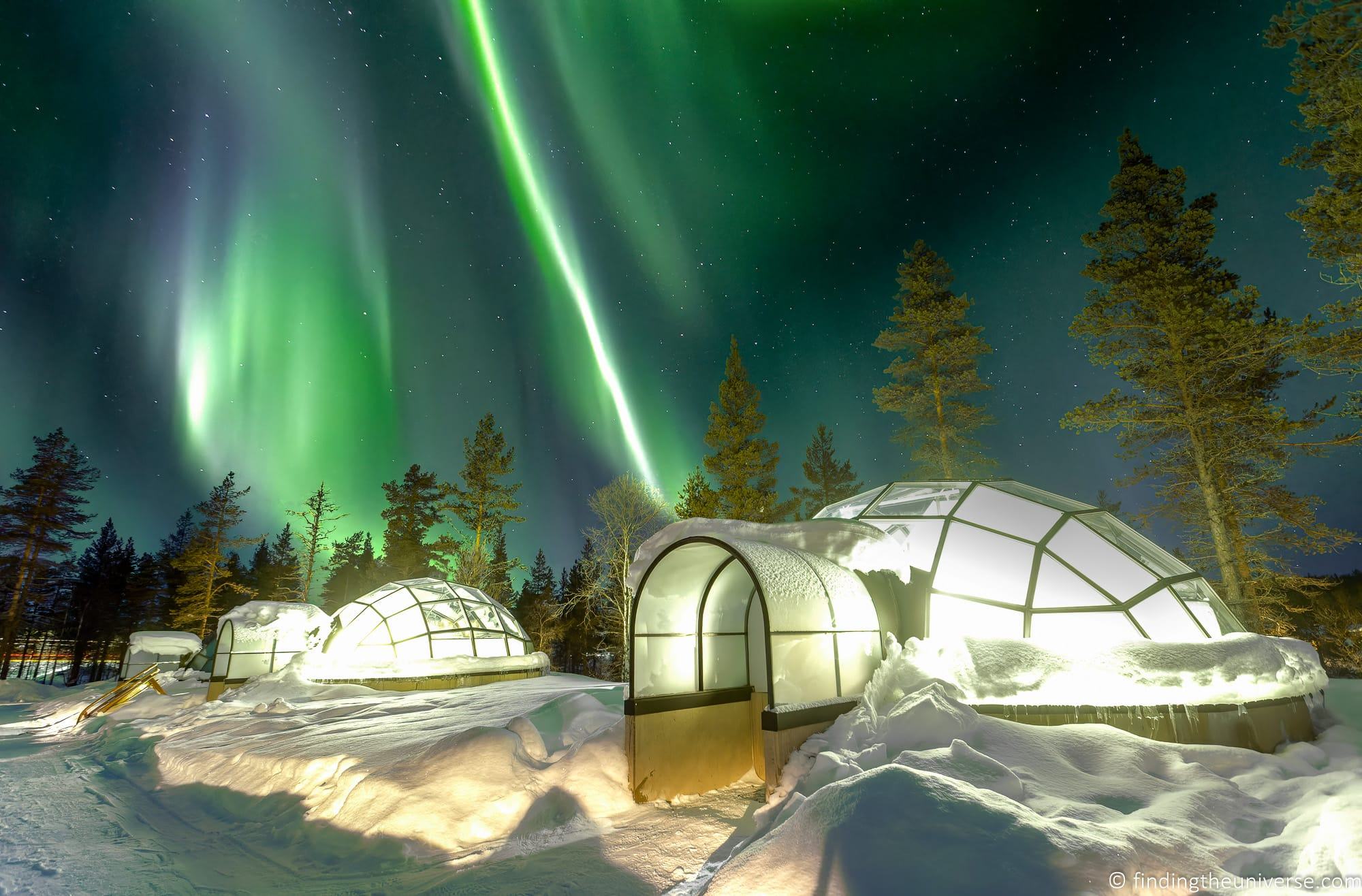The nighttime scene captures the ethereal beauty of the Aurora Borealis in a snowy, Northern landscape. The sky is alive with twinkling stars and vibrant, wavy streaks of green and purple that paint the heavens with a breathtaking display. The ground is blanketed in shimmering snow and ice, which reflects the colorful sky above. In the foreground, a small cluster of white, igloo-like domes, possibly accommodations for tourists, are arranged in a neat row. These domes have well-shoveled pathways leading to their entryways, and they glow warmly from within, suggesting the presence of lights or lamps inside. The structures are primarily white with some black borders and patterns, and their bases appear to be made of a tannish-brown material, possibly cement. Tall pine trees frame the scene, adding to the serene, wintry ambiance. A watermark at the bottom corner reads "findingtheuniverse.com," adding a touch of authenticity to this magical view.